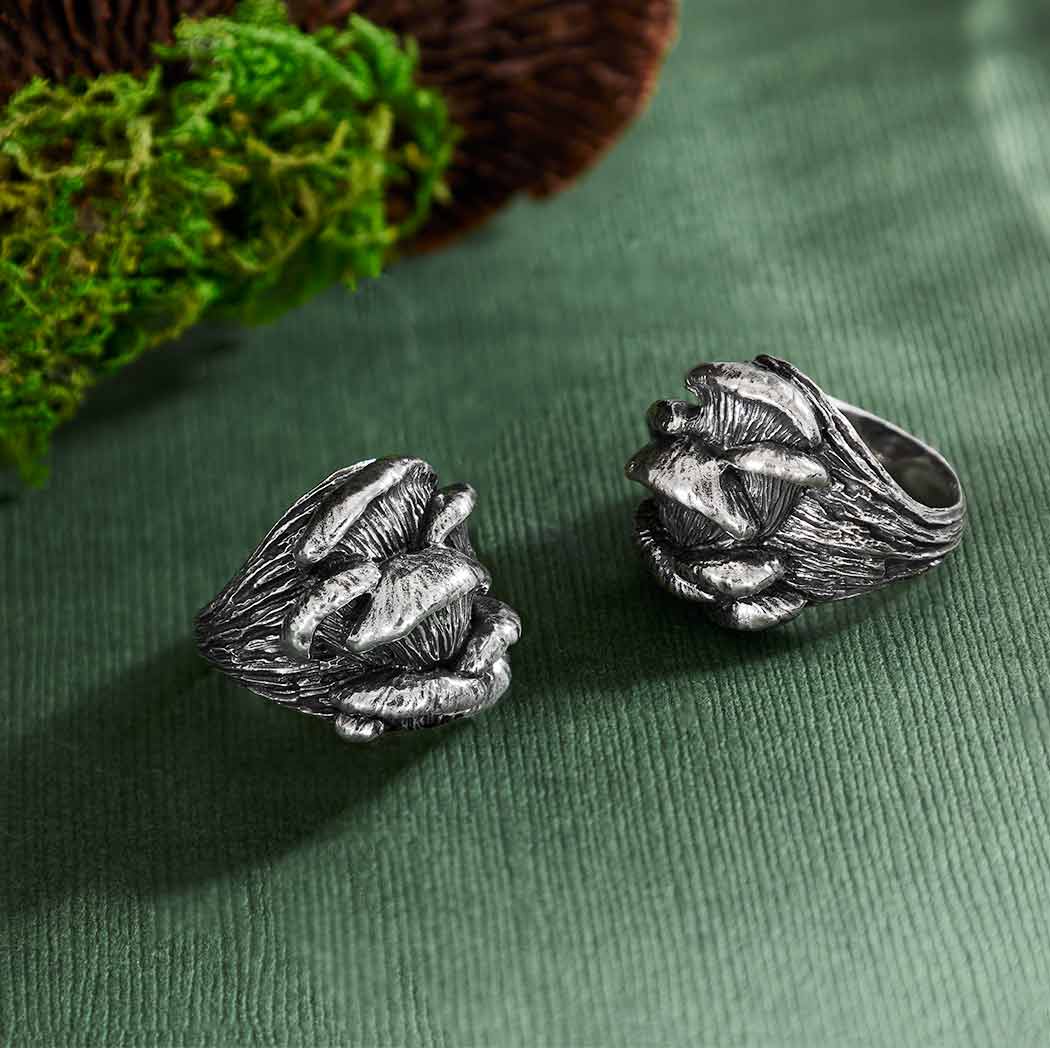In this detailed close-up photograph, the focal point is two silver rings adorned with intricate mushroom designs. The rings are situated on a textured, green ribbed surface, possibly a tablecloth, accompanied by a bit of greenery in the background, hinting at an amplified view of a plant. The larger of the two rings has a prominent mushroom cap design, with grooves mimicking the gills found on the underside of a real mushroom. The base of this ring features multiple smaller mushroom figures, creating a textured and organic pattern. The underside of the ring, the band that wraps around the finger, exhibits a striped, grooved appearance, adding to its intricate craftsmanship. The overall composition, with the silver hues contrasting against the green backdrop, makes for a visually striking image. The green and brown elements seen to the top left add to the natural ambiance of the setting.